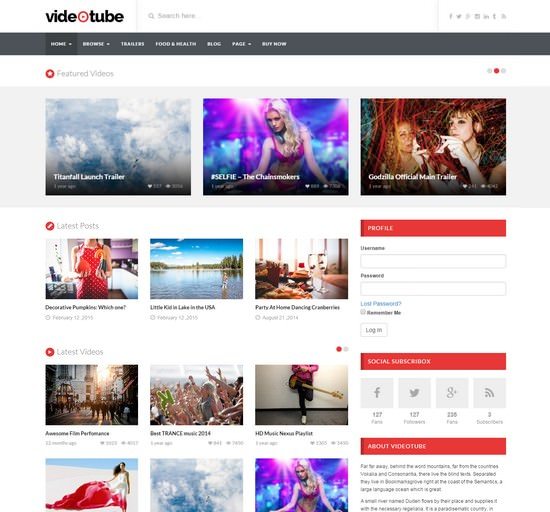The screenshot captures a section of the "VideoTube" website. At the top of the page, "VideoTube" is prominently displayed in black text, with a distinctive "O" styled as a red bullseye featuring a red dot in its center. To the right, there is a search bar labeled "Search Here," accompanied by various social media icons. Beneath this header, a dark gray to black gradient banner spans horizontally, containing navigation options: Home, Browse, Transfers, Food and Health, Blog, Page, and In Buff Now (with blurred, difficult-to-read text).

Below the banner, against a white background, there is a red circle with a white star inside it, next to the heading "Featured Videos." The featured section is outlined by a light gray background at the top, showcasing three videos displayed side by side. Further down, there is a section labeled "Latest Posts" on a white background, listing three posts side by side at the top.

The middle section highlights "Latest Videos," featuring six different video thumbnails. Towards the right side of the page, there's a user profile section with fields labeled: Profile, Username, Password, Lost Password, Social, Subscribe Box, followed by details about the site, "About VideoTube."